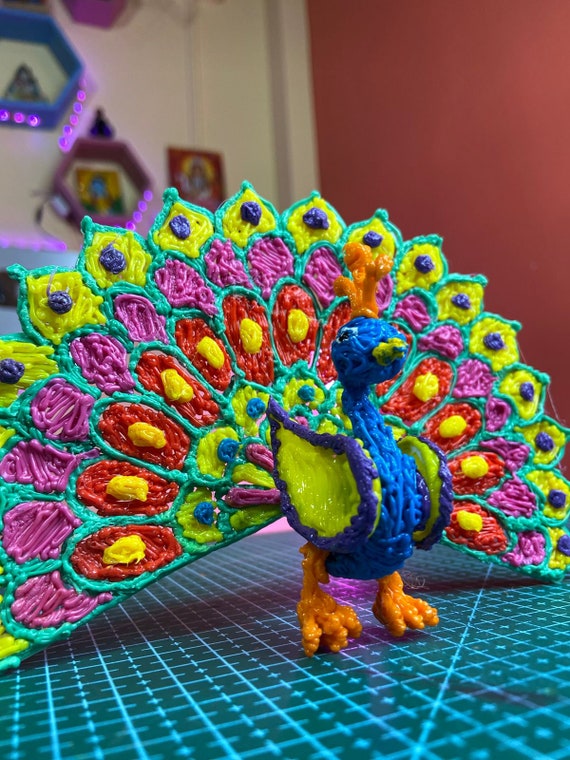The image depicts a detailed 3D craft of a peacock, likely made from pieces of plastic or a similar material. The peacock has a blue body with orange feet and a small tuft on its head. Its wings are primarily yellow with hints of blue, and the peacock's elaborate tail feathers are a vibrant mix of colors. The outermost layer of the feather arrangement is teal, with subsequent layers showing a variety of colors including yellow with blue dots, red with yellow dots, and sections of pink, lime green, and purple with dark purple dots. The peacock is positioned on a tabletop that appears black with blue lines, resembling a graph or design surface. In the background, the left wall is a rosy red, and the right wall is white, featuring hexagon-shaped wall shelves, some holding pictures. The scene is slightly blurred, highlighting the crafted peacock as the focal point.